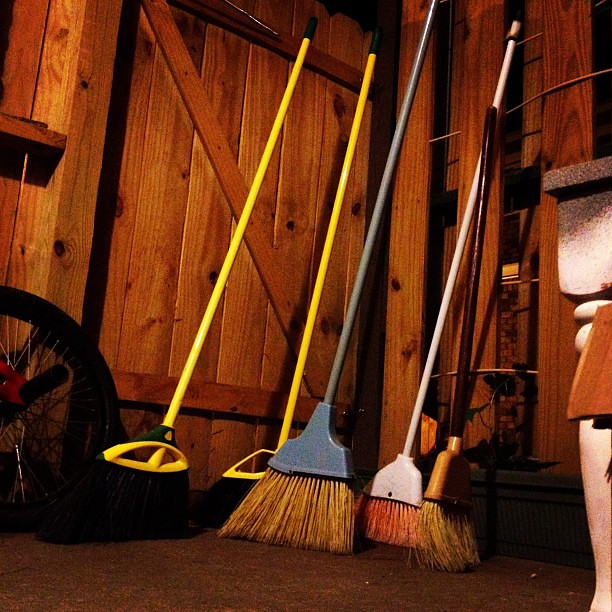This photograph captures the quaint interior of a well-crafted wooden shed. The focal point is a collection of five brooms standing upright in the corner, set against walls and a door made of finely stained vertical wooden planks. The two brooms on the far left feature yellow handles and black bristles, lending a uniform appearance. Moving towards the right, the next broom has a grey handle paired with brown bristles. Another broom, with a white handle and brownish-reddish bristles, stands nearby, followed by a broom with a black handle and brown bristles at the far right. The well-finished woodwork, which includes a door with vertical planks supported by horizontal beams at the top and bottom and a diagonal brace, adds a rustic charm to the setting. Additional details in the image include a bicycle wheel at the bottom left and the legs and edge of a sink barely visible on the right side.